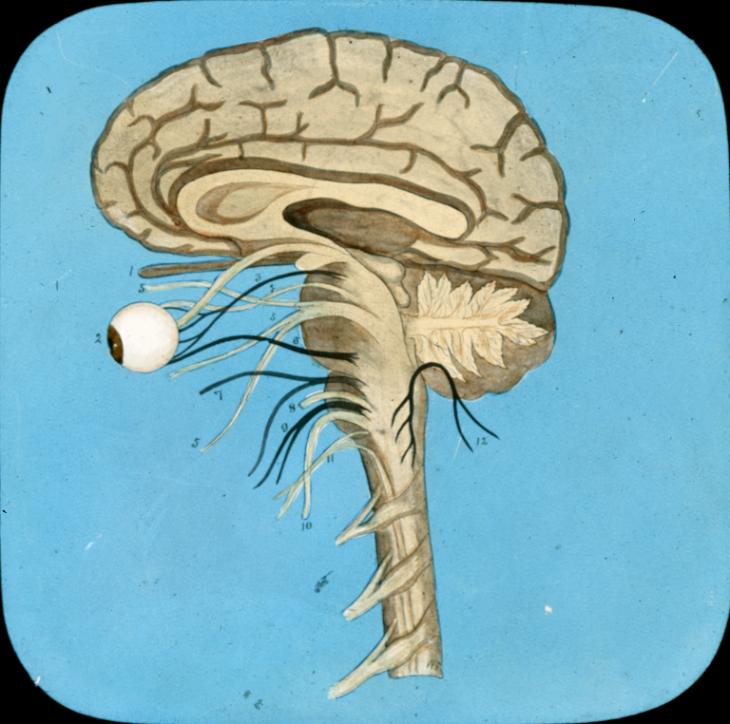This image features a detailed side cutaway view of the internal structures of a human head, from the brain extending down to the neck. Displayed against a blue background, this digital artwork or sketch comprises beige, brown, and black hues to depict a realistic and informative illustration. The notable components include a segmented brain connected to the spinal cord, with prominently displayed veins or arteries. One eye is distinctly present, positioned as if the skull's face were turned to the left, revealing the eyeball's white sclera, black pupil, and brown iris. Additional elements, such as a leaf-like structure appearing to originate from beneath the brain, add a surreal dimension to the illustration. This educational image, potentially used for teaching medical students or nurses, incorporates numbered labels on various parts, likely referencing textbook annotations to facilitate the learning of anatomical terminology. The blue background enhances the vivid depiction of the inner head structures, evoking an underwater ambiance, further emphasizing the clear and meticulous representation of the brain, eyeball, and spinal cord within the half-sectioned skull.